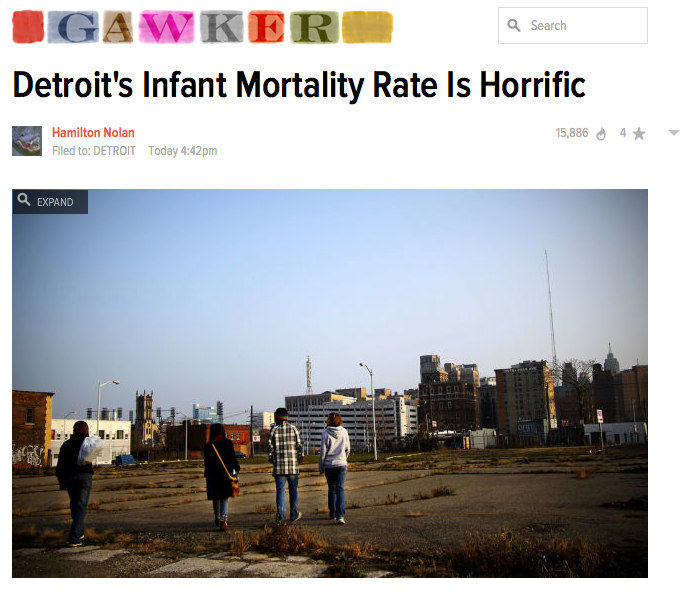The image, sourced from Gawker, presents a stark visual narrative under the headline "Detroit's Infant Mortality Rate is Horrific" by Hamilton Nolan, posted today at 4:42 PM with a view count of 15,886 and a rating of four stars. In the foreground of this digital article layout, a photograph captures a desolate scene: four individuals—likely two men and two women—stand with their backs to the camera, possibly engaged in conversation, as they face an expansive, barren lot scattered with dark greenery, weeds, and cement slabs. The lot gives way to a distant, yet more intact array of buildings no taller than ten stories. Above, the sky is a clear, vibrant blue, bereft of clouds, setting a stark contrast to the grim, run-down foreground. The upper section of the image includes a Gawker header, formatted in colorful, shaded boxes spelling out "Gawker," alongside a search bar. The setting perhaps alludes to a juxtaposition between urban decay and potential revitalization, highlighted by the distant, seemingly better-maintained cityscape the individuals appear to be heading toward.